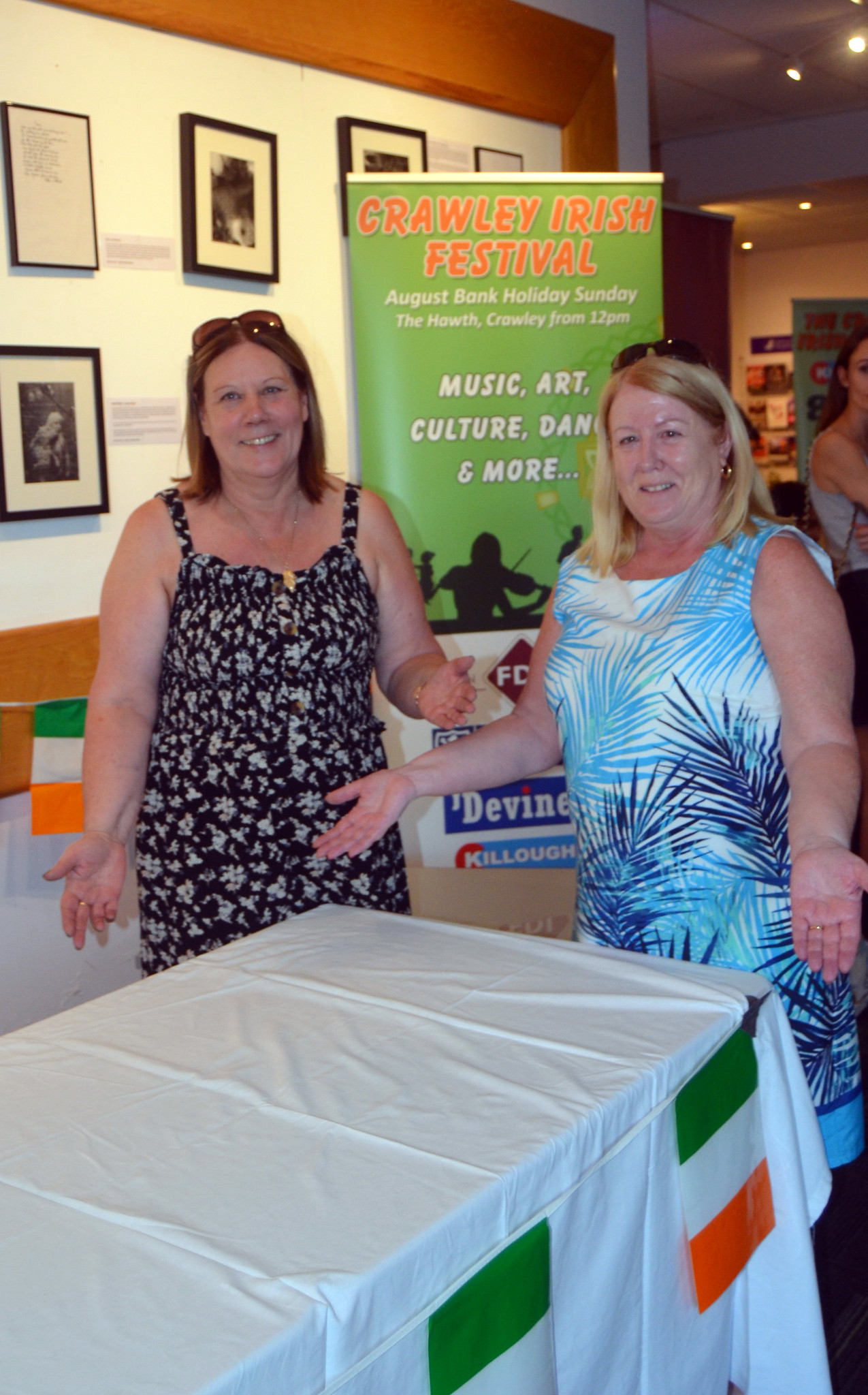This detailed color photograph captures two women standing behind a table adorned with a white tablecloth featuring several small Irish flags in green, white, and orange. Both women, who appear to be Caucasian and possibly siblings, are smiling at the camera while holding their hands out over the table, palms up. The woman on the right has blonde hair and is dressed in a blue and white summer dress, while the woman on the left has dark hair and is wearing a black and white summer dress. Both have sunglasses perched on their heads. A prominent green sign situated between them reads "Crawley Irish Festival" in bold red letters, with additional white text below it announcing "August Bank Holiday Sunday," and "Music, Art, Culture, Dance, and More." The scene is set against a white wall with framed photos, suggesting an indoor venue. A partial figure of another individual is visible in the upper right corner, adding to the bustling atmosphere of what appears to be a lively event.